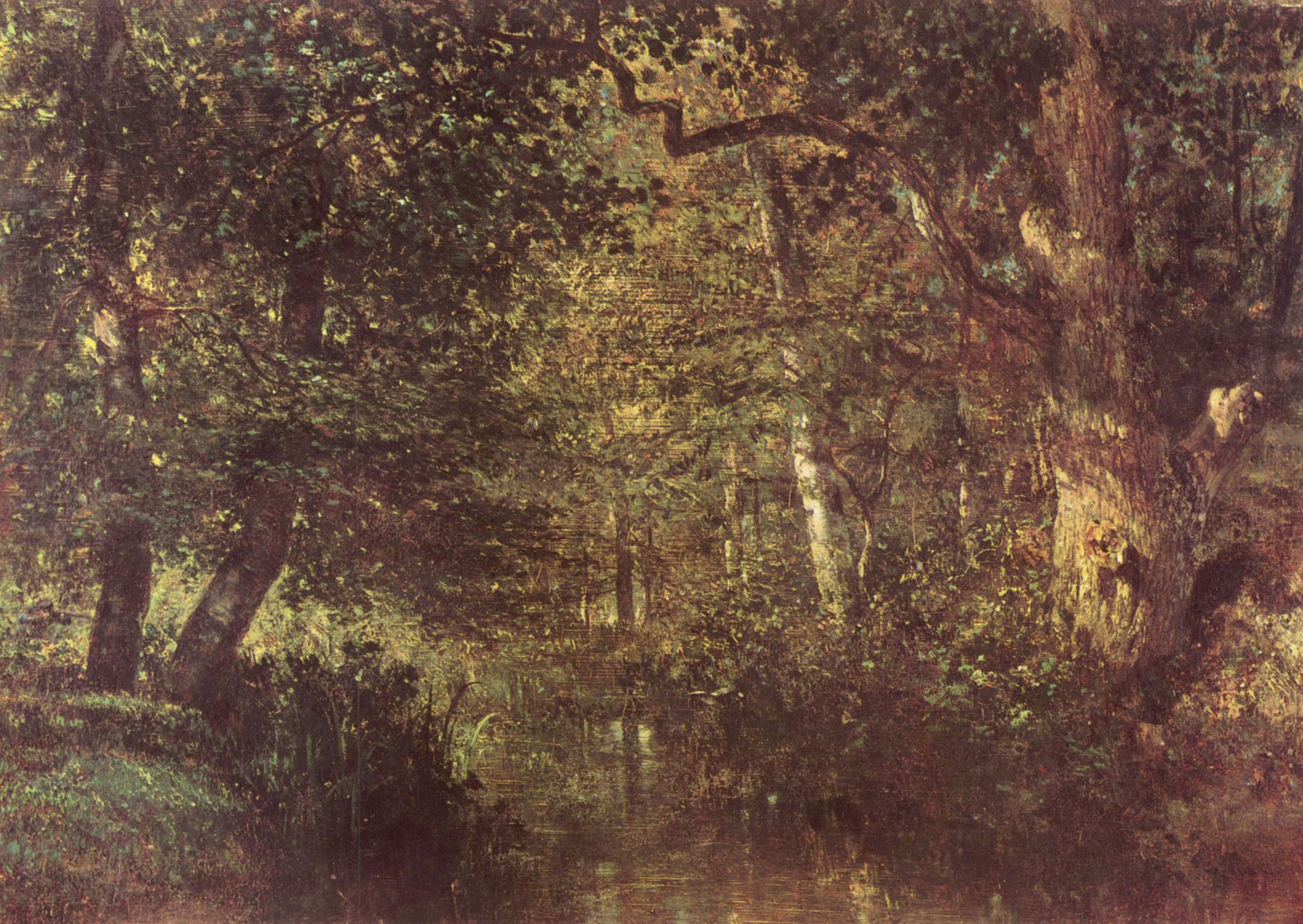This is a highly detailed and realistic painting of a serene forest scene, almost photographic in its precision, possibly created with oil or acrylic paints. The composition features a small, smooth, slightly rippled creek running through the center, bordered by lush, vibrant shades of green, yellow, and earthy brown. On the right side, there is a thick tree trunk bathed in golden sunlight, with wiry branches and green leaves at the top. On the left side, two smaller trees grow from a hill, their trunks adding to the intricate layering of the natural landscape. The scene has an impressionistic feel, reminiscent of works by Monet or Degas, and evokes a tranquil, sunny yet slightly overcast day in the woods.